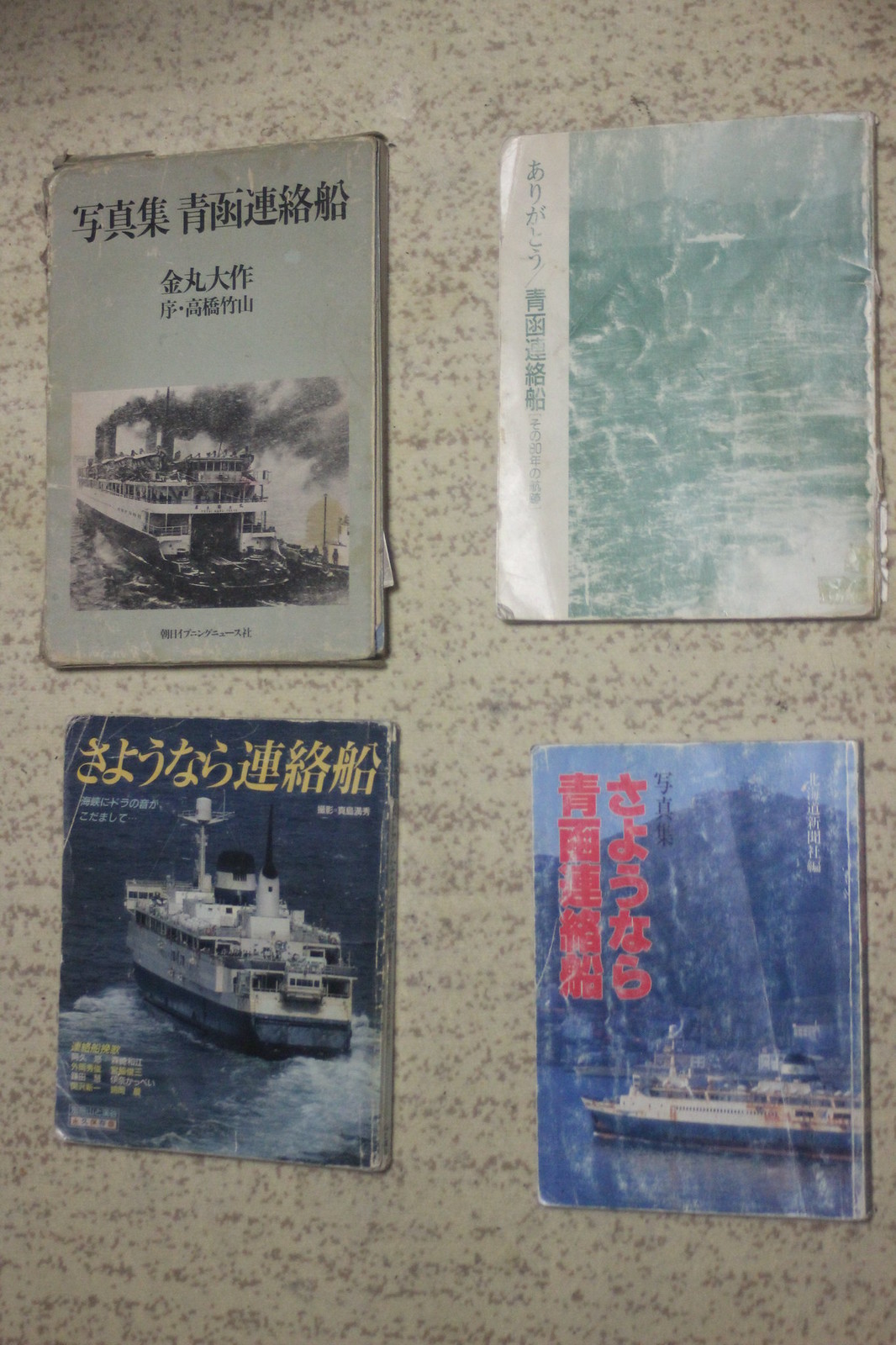A photograph captures four tattered and vintage pamphlets or thin books, written in Japanese, laid out on a mottled, grey, formica countertop. The top left pamphlet has a worn, grey cover featuring a black-and-white image of a steamboat with black smoke billowing from its stacks. To its right, the top right pamphlet has a light blue, heavily crinkled and faded cover, depicting open water and possibly distant land, with Japanese writing down the left side. The bottom left pamphlet displays a more modern-looking large ship on a dark blue sea, with white waves trailing behind, and Japanese text in yellow across the top. Finally, the bottom right pamphlet, also worn and marked with creases, shows a side view of a white ship against a backdrop of hills or mountain ranges, with vertical Japanese writing in red along the left-hand side. Each pamphlet’s aged and fragile state hints at their long history, possibly related to maritime travel.